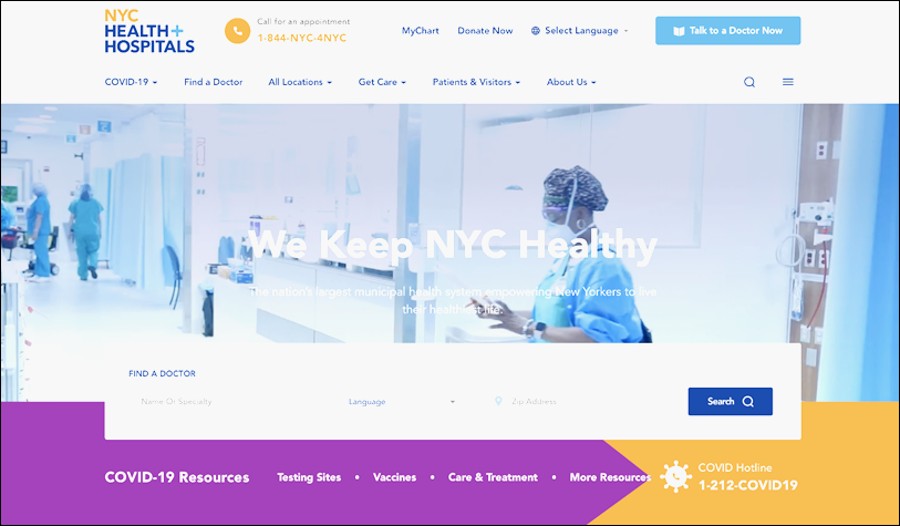Homepage of NYC Health + Hospitals:

The NYC Health + Hospitals homepage prominently features a large, somewhat overexposed image of three healthcare professionals inside a hospital setting. These individuals are dressed in scrubs, wearing hairnets, and face masks, emphasizing a sterile and professional environment. Despite the slight fogginess of the image, the foreground elements are clear and detailed.

At the top of the page, the NYC Health + Hospitals logo is displayed. Next to the logo is a yellow circle containing a phone handset icon, accompanied by the text "Call for an Appointment" followed by a contact phone number.

Below the header, there are several navigation buttons:
- **MyChart**
- **Donate Now**
- **Select Language** (with a dropdown menu for language options)
- A large light blue rectangle labeled "Talk to a Doctor Now," featuring an icon of an open book.

Further down the page, additional navigation options include:
- **COVID-19** (with a pop-up menu)
- **Find a Doctor**
- **All Locations** (with a pop-up menu)
- **Get Care**
- **Patients and Visitors**
- **About Us**

This detailed layout provides users with convenient access to various services and information offered by NYC Health + Hospitals.